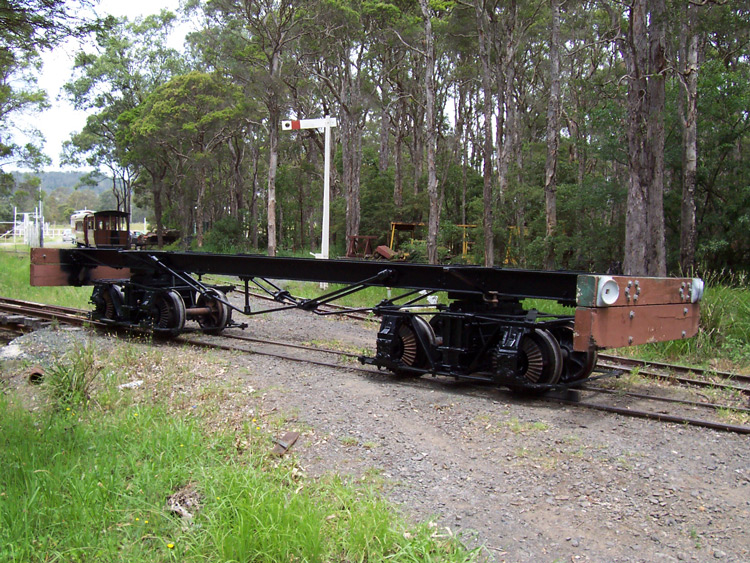This photograph captures a rustic, seemingly vintage scene of a stripped-down, flatbed-style train cart situated on a railway track amidst a sylvan backdrop. In the foreground, a patch of green grass transitions into gravel strewn with dark gray, gray, light brown, and orange pebbles leading up to the rails. The flatbed train cart, devoid of any superstructure, is predominantly black and gray with hints of red and brown, and prominently displays its undercarriage with eight black wheels and an array of mechanical components. Sharing the foreground, another train cart, possibly intended for passengers, becomes partially visible. The background reveals a scenic forest with towering trees, their tops cropped by the image, suggesting the lushness of summer or spring. A white post, equipped with a perpendicular arm adorned with white, red, and a dot on its tip, stands out amid the greenery. Additional details include a white sign and some kind of distant white gating, all contributing to the photograph's nostalgic and vintage ambiance.